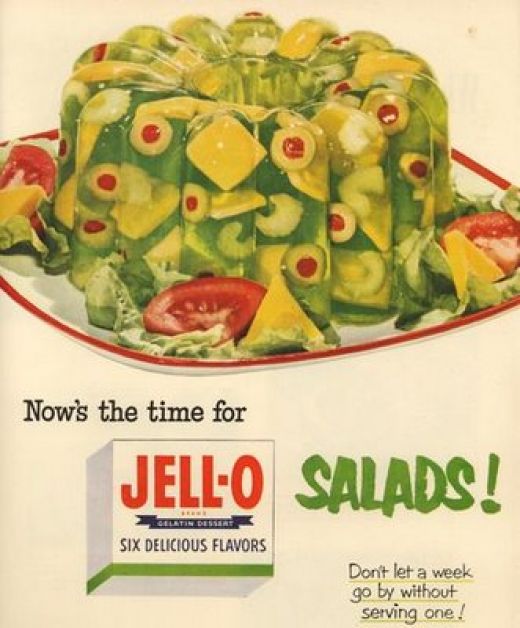This vintage advertisement from the mid-20th century features a Jell-O salad, prominently displayed against a cream-colored background. The eye-catching image shows a Bundt cake-shaped mold of lime green Jell-O, studded with pimento-stuffed olive slices, celery pieces, and possibly cheese or avocado. Surrounding the Jell-O mold is a garnish of crisp lettuce, tomato wedges, and lemon pieces, creating a colorful, if unconventional, presentation. At the bottom, the ad boldly proclaims in green lettering, "Salads!" followed by, "Don't let a week go by without serving one." An additional tagline reads, "Now's the time for Jell-O," highlighting the six delicious flavors available, encapsulated visually by a white Jell-O box with red letters and a distinctive green band.